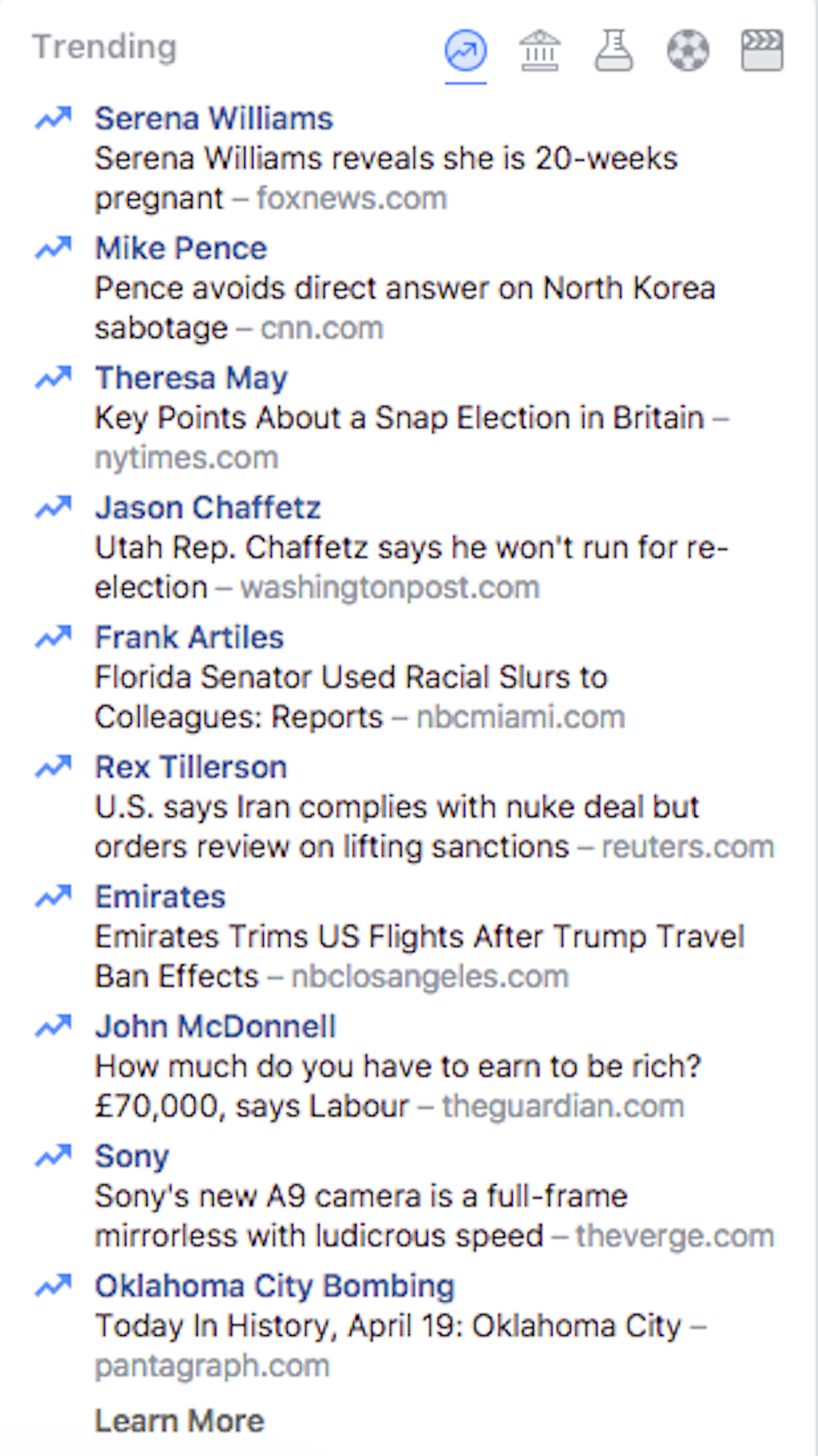**Caption:**

A comprehensive screen grab illustrating the top trending news articles across various categories including science, politics, sports, and entertainment. The page header prominently displays "Trending," accompanied by icons signifying different news sections. There are ten trending news stories listed:

1. **Serena Williams:** "Serena Williams Reveals She is 20 Weeks Pregnant" - FoxNews.com
2. **Mike Pence:** "Pence Avoids Direct Answer on North Korea Sabotage" - CNN.com
3. **Theresa May:** "Key Points About a Snap Election in Britain" - New York Times.com
4. **Jason Chaffetz:** "Utah Representative Chaffetz Says He Won't Run for Re-election" - WashingtonPost.com
5. **Frank Artiles:** "Florida Senator Used Racial Slurs to Colleagues" - NBCMiami.com
6. **Rex Tillerson:** "US Says Iran Complies With Nuke Deal but Orders Review on Lifting Sanctions" - Reuters.com
7. **Emirates:** "Emirates Trims US Flights After Trump Travel Ban Effects" - NBCLosAngeles.com
8. **John McDonnell:** "How Much Do You Have to Earn to be Rich? 70,000 Euros, Says Labour" - TheGuardian.com
9. **Sony:** "Sony's New A9 Camera is a Full-frame Mirrorless With Ludicrous Speed" - TheVerge.com
10. **Oklahoma City Bombing:** "Today in History, April 19th: Oklahoma City" - Pantagraph.com

Additionally, there's a link at the bottom to explore more articles.